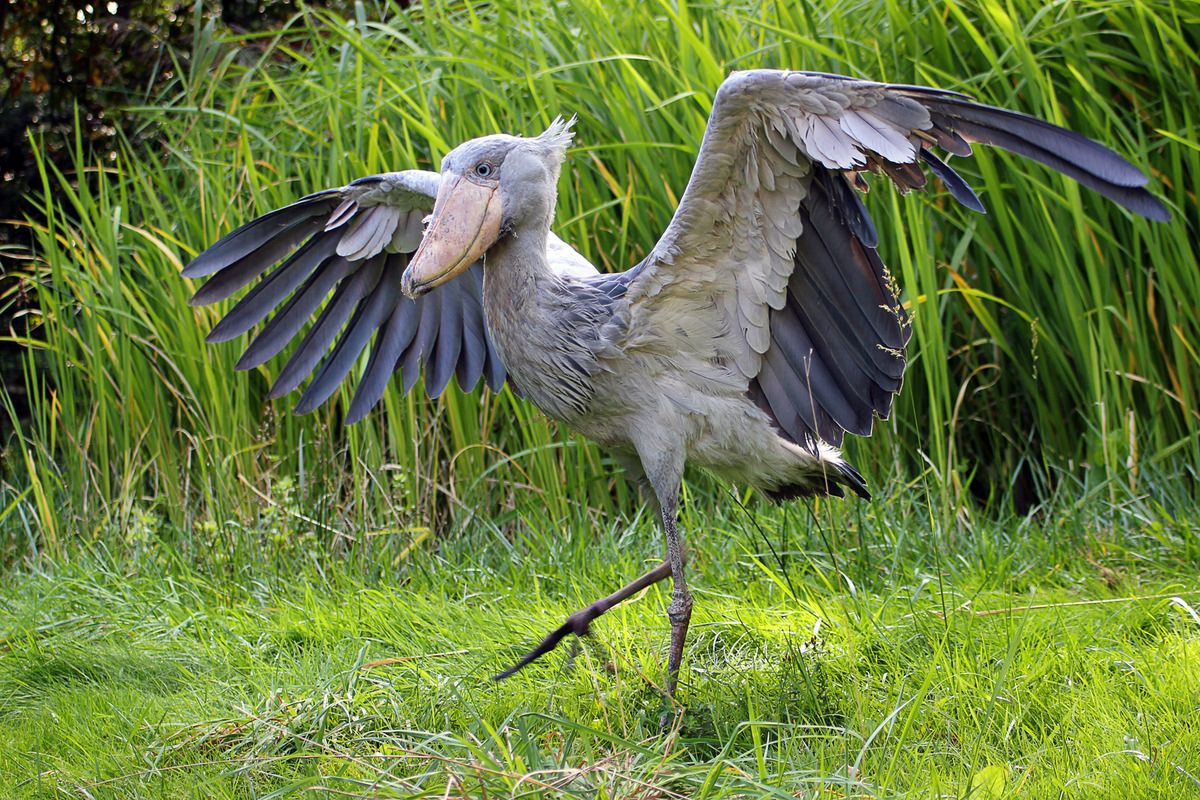In a natural setting filled with lush greenery, this striking bird commands attention as it strides across a patch of short, rugged grass. The foreground grass, a couple of inches high, gives way to an imposing expanse of tall grass, which reaches several feet in height and appears wild and unmaintained. In the distance, dense, dark foliage obscures the sunlight, creating a shadowy backdrop that adds to the scene's depth. 

Dominating the scene is the bird itself, reminiscent of a stork but with distinct features more akin to a pelican. Its body, cloaked in light gray feathers, is large and robust, contrasted by its exceedingly long, thin legs that end in long toes. These legs are darker in color and have noticeable knee joints, resembling the anatomy of a stork. 

The bird’s expansive wings, currently outstretched, showcase a dichotomy of colors: the upper surfaces are light gray, while the underside feathers take on a dark blue hue. This display reveals a wingspan that is impressively broad. Its neck is elongated and a light bluish-gray, leading to a large head adorned with a few pointy feathers at the back. The head itself is light blue, and it features distinct blue eyes and a large, banana-yellow beak, completing its majestic appearance. The bird's posture as it walks and spreads its wings might suggest a moment of asserting its presence or preparing for flight. Overall, the scene raises curiosity about the bird's authenticity, with some aspects of its vivid coloration and grandeur leading to speculation that it might be a highly detailed 3D model or an expertly crafted Photoshop creation.